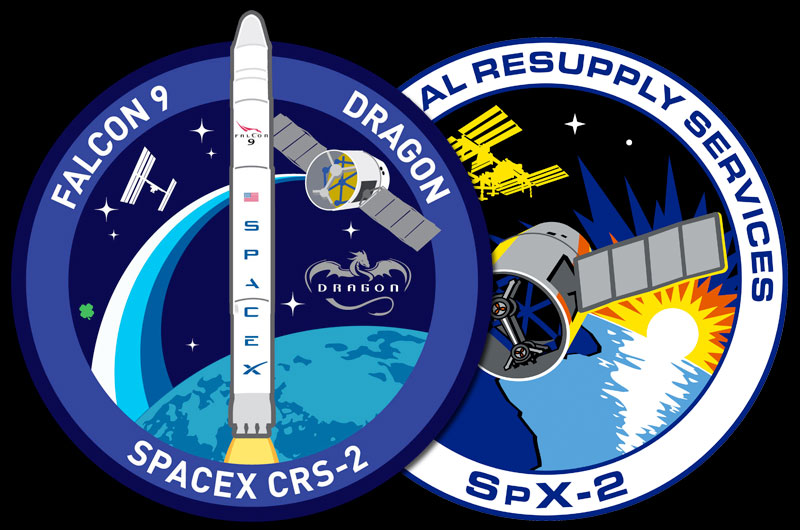The image features two overlapping logos set against a black background, both emblematic of SpaceX missions. The upper logo is predominantly blue and circular, with the words "Falcon 9 Dragon" inscribed in white across the top and "SpaceX CRS-2" at the bottom. Encircling these inscriptions is a medium blue border, which is further surrounded by a navy blue rim. Central to this logo is a dynamic illustration of a tall, white rocket launching, flames billowing from its engines. The rocket is branded "SpaceX" and also displays the American flag and the label "Falcon 9" towards its nose. Adjacent to the rocket is a depiction of a satellite. Overlaying the rocket image is an artistic dragon design with the name "dragon" boldly written across it. Surrounding the rocket and satellite are various stars and a subtle four-leaf clover on the left, adding an element of luck to the design.

The second, slightly obscured logo beneath the first, also has a circular structure with a white inner border and a navy blue outer edge. The top of this emblem contains the words "Commercial Resupply Services," while the bottom features "SPX-2." The central image within this logo shows a radiant sunburst rising over a body of water, creating a shimmering reflection. A satellite with distinctive gray panels occupies the foreground, with additional yellow satellites situated in the background, enhancing the celestial theme of the design.